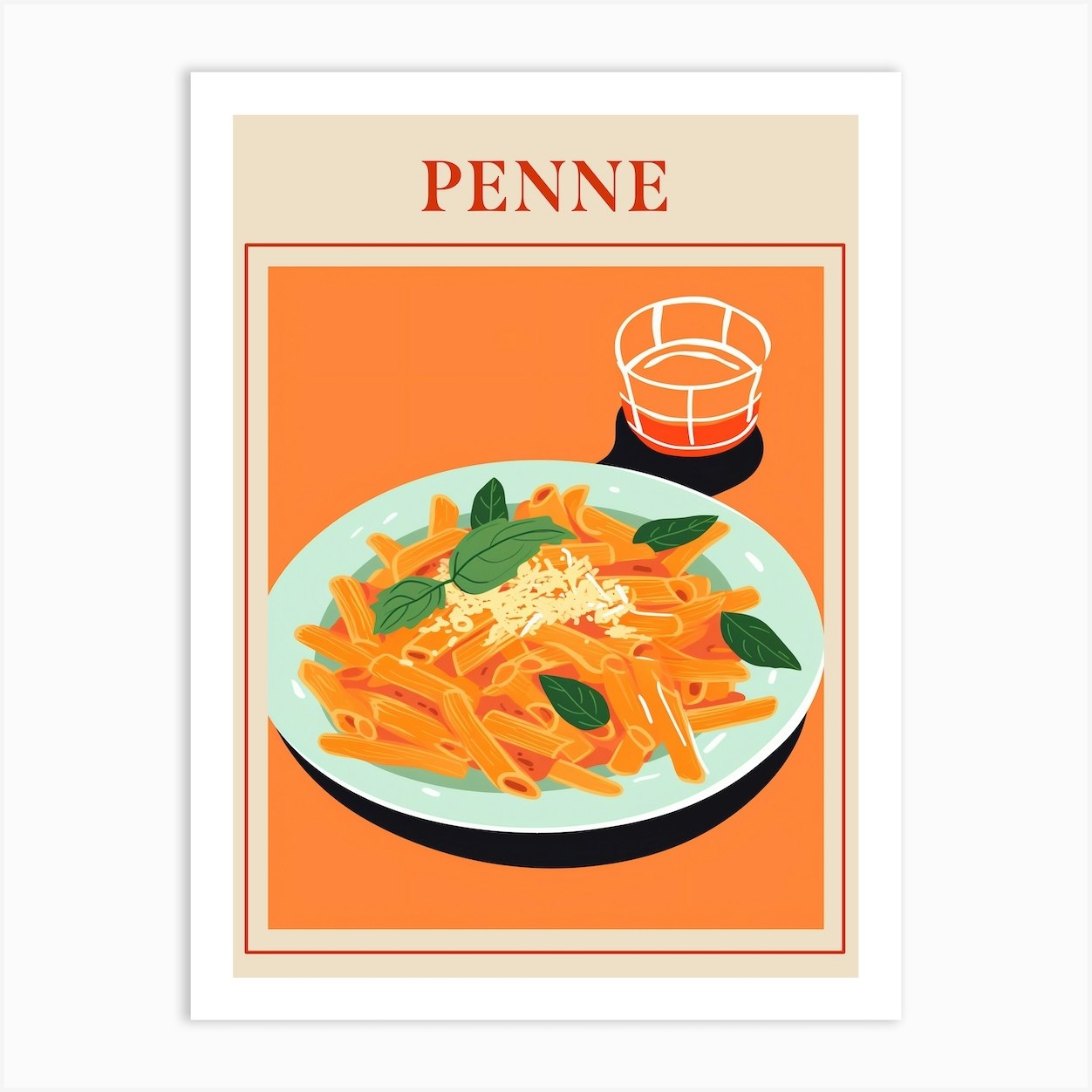This image depicts a product photograph showcasing a minimalist, modern poster designed to advertise food. The poster itself is presented on a light gray background, creating an illusion that it is floating in an empty void. It features a substantial white border framing the poster, which has a tan-colored background.

At the top of the poster, in large, bold, uppercase orange letters, is the word "PENNE" spelled out as P-E-N-N-E. Below this text, the central focus of the poster is an orange rectangle bordered by a thin orange line and a thinner tan line. Inside the orange rectangle, there is a stylized, digitally drawn image of a plate of penne pasta. 

The plate is white, round, and piled with light orange penne pasta, topped with green basil leaves and a sprinkling of what appears to be Parmesan or Romano cheese. The plate casts a distinct shadow toward the lower right edge. Positioned just above the plate, at approximately the 1 o'clock position, is a white outline drawing of a half-full glass, which casts a similar shadow to the lower right. 

The sophisticated yet simple design, with its clear focus on the food illustration and clean typography, makes this poster an eye-catching piece for any modern kitchen or dining area.